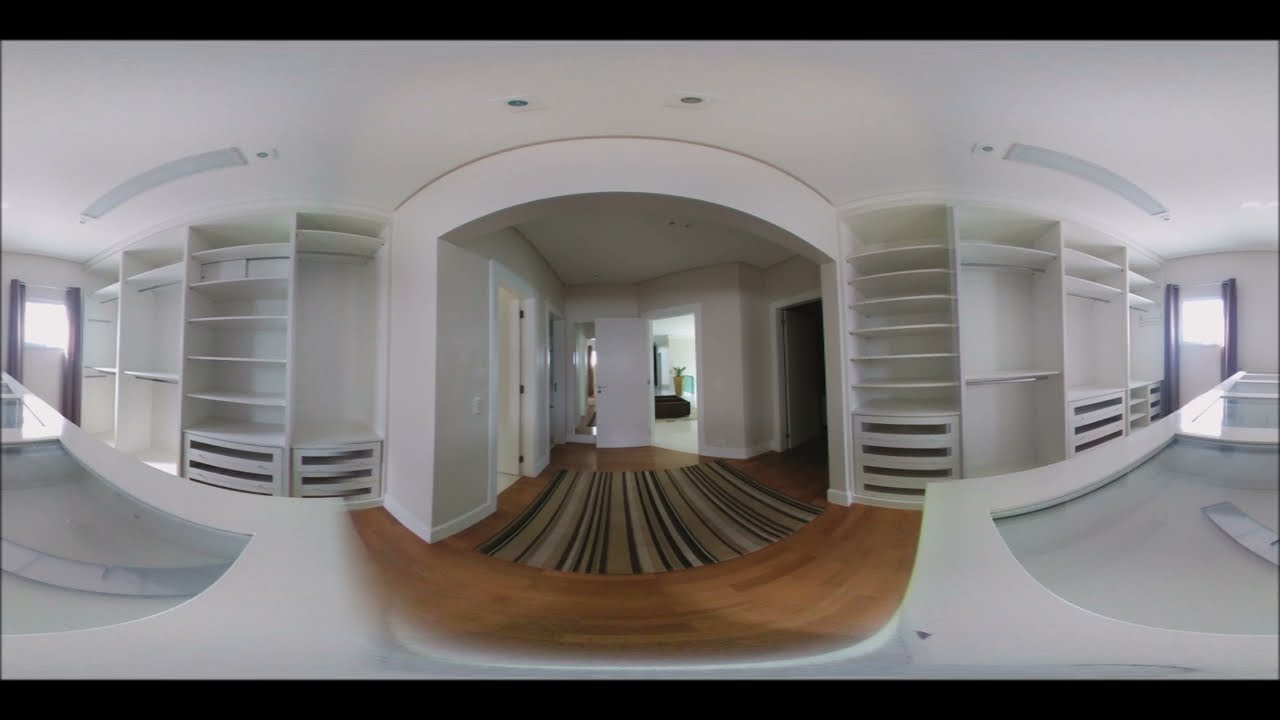The image features a business logo and contact information against a gradient background that transitions from white at the top to light gray at the bottom. Central to the image is a blue circular logo with white wavy lines and a dark shadow on its right side. Positioned below the logo in black font are the words "J. Almeda Matos." In blue font beneath that, it reads "NEGÓCIO IMOBILIÁRIO LTDA." Following this, in smaller black font, is the identifier "CRECI: 16252-J". Below the CRECI number, additional information is provided in black font: contact numbers "5511 4195-5988" and "5511 7889-1260," and the address "Calçadas das Anémonas, 155, Central Comercial Alpha Bill, Barueri, SP." The image also lists two websites: "www.jalmeidamatos.com.br" and "www.jalmeidamiami.com."